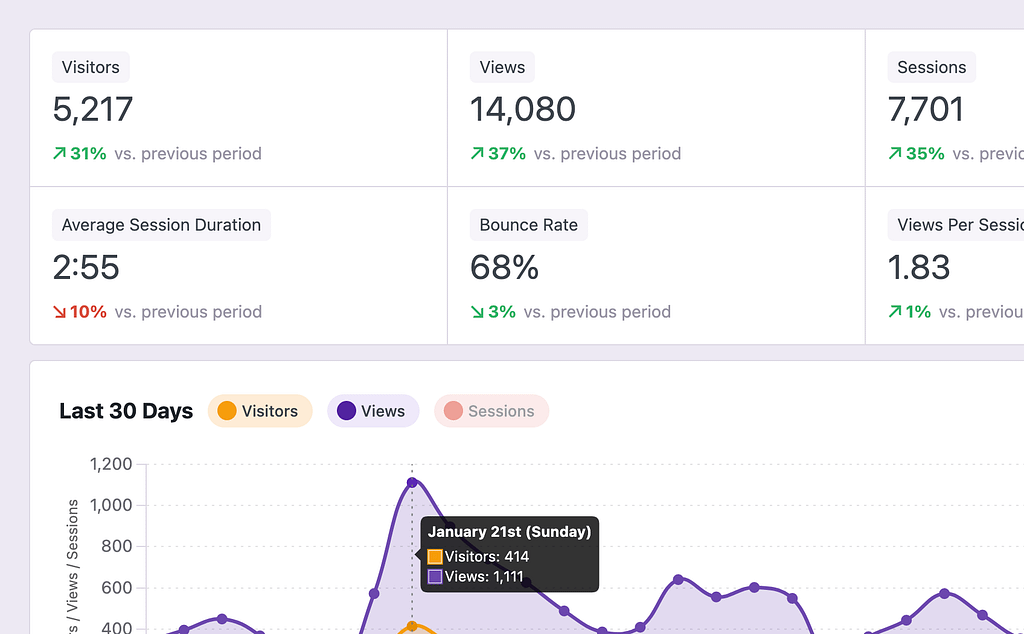The image is a screenshot capturing the top-right segment of an online dashboard. It features a layout that's slightly wider than it is tall, with a thin border that transitions from a light gray to a purplish hue running down the left side. About halfway down this edge, another similar border runs horizontally across but fades as it reaches the right side, indicating that only the upper left section of the dashboard is visible.

In the top-half section of the screenshot, there are six distinct squares arranged in two rows of three. These present various metrics starting with "Visitors," "Views," and "Sessions" in the top row, each accompanied by a numerical value. Beneath each of these, there's an indicator for percentage change compared to the previous period, represented by a green percentage figure and an upward arrow when the metric is trending positively.

The second row of squares continues with "Average Session Duration," "Bounce Rate," and "Views Per Session," each displaying their corresponding figures along with percentage changes from the previous period, similar to the top row.

Below these squares, part of a chart is visible, though some of it is cut off at the bottom. This chart is titled "Last 30 Days" and includes data points marked with orange for "Visitors," purple for "Views," and a lighter orange for "Sessions." The chart itself shows trends over the past 30 days, with lines fluctuating up and down to reflect changes in views per session metrics, but crucial details at the bottom of the chart remain obscured in the screenshot.